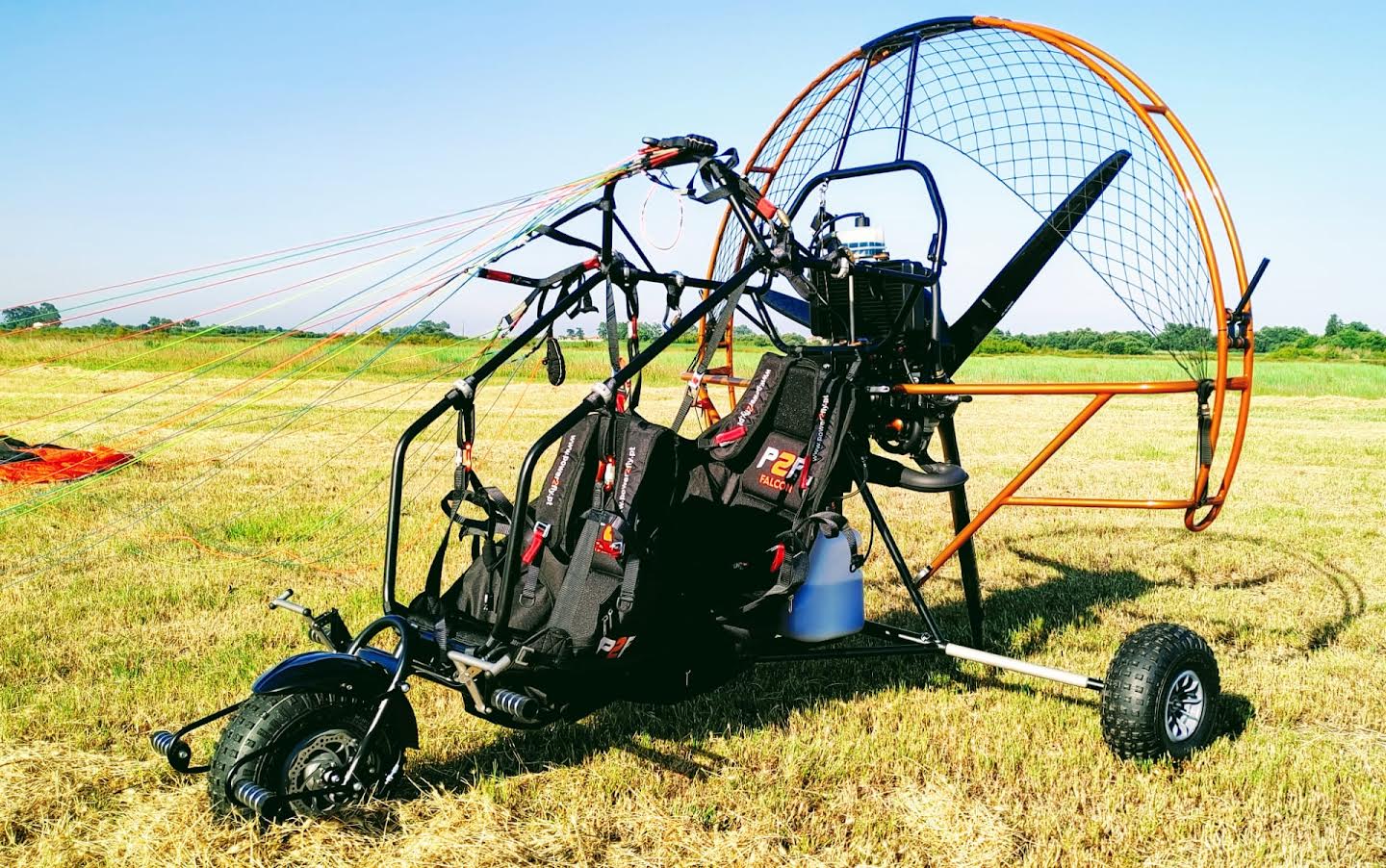The image depicts an open-air, three-wheeled vehicle designed for flying using a parachute for wings, typically known as a powered parachute. The vehicle features two black seats equipped with five-point safety harnesses, positioned one behind the other. The frame of the vehicle is exposed, providing no enclosure for the occupants. At the back of the vehicle, there is a prominent engine housed within a burnt orange, double-layered cylindrical metal cage, akin to those found on airboats, to protect against the rotating twin black propellers. The vehicle is currently parked on grass under a bright turquoise sky, bordered by trees with green treetops in the background. The front part of the vehicle has an array of multicolored strings leading to the open parachute, which is intended to be airborne while driving and neatly folded upon landing. The wheels are rubber with black tires and silver hubcaps, and the rear axle is notably long and narrow to support the motor assembly.